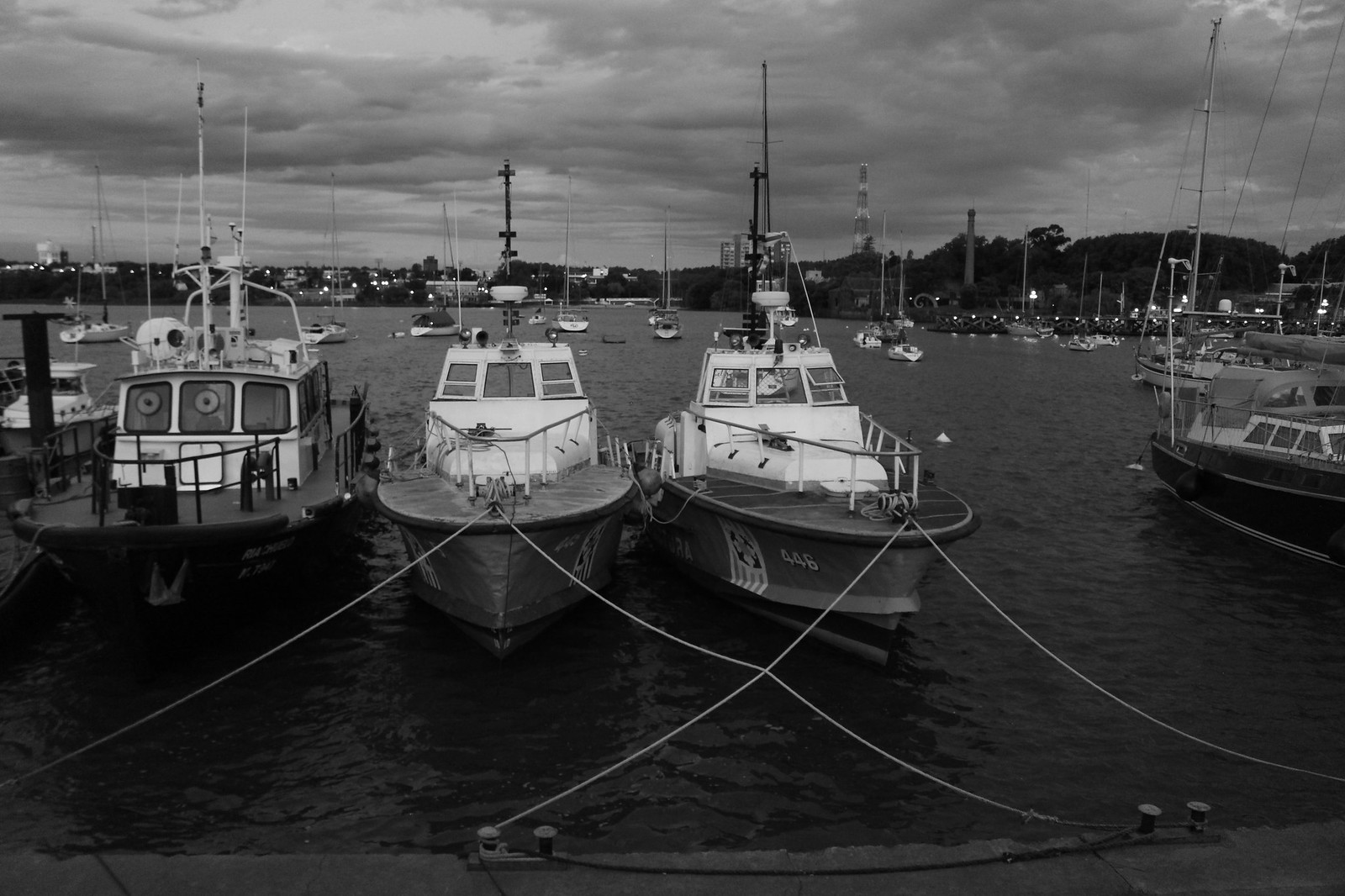In this black and white photograph, a marina is depicted on a cloudy day, with overcast skies filled with puffy clouds that cast a subdued, somber light onto the scene. The image captures a horizontal expanse primarily showcasing the waterfront and boats, framed by distant rolling hills and a tree line that suggests a lush, verdant backdrop, indicative of a tropical region during spring or summer months. 

In the background, beyond the water, one can glimpse faint city lights twinkling through the gloom, signaling an urban area nestled beyond the shoreline. Amidst this setting, numerous boats are moored. Smaller schooners and fishing ships float in the water, detached and serene, with no sails hoisted. 

In the foreground, occupying the left and center-right portions of the frame, three prominent boats are tied up at the dock with sturdy white ropes looped around metal posts. These boats, possibly utility or emergency vessels, each feature distinctive cabins brimming with antennas. One particularly notable boat in the center-right bears the number "446" emblazoned in white on its side, and they collectively add a layered complexity to the composition. The dock's edge is just visible at the bottom of the photo, anchoring the scene in a tangible reality against the ethereal water and sky.